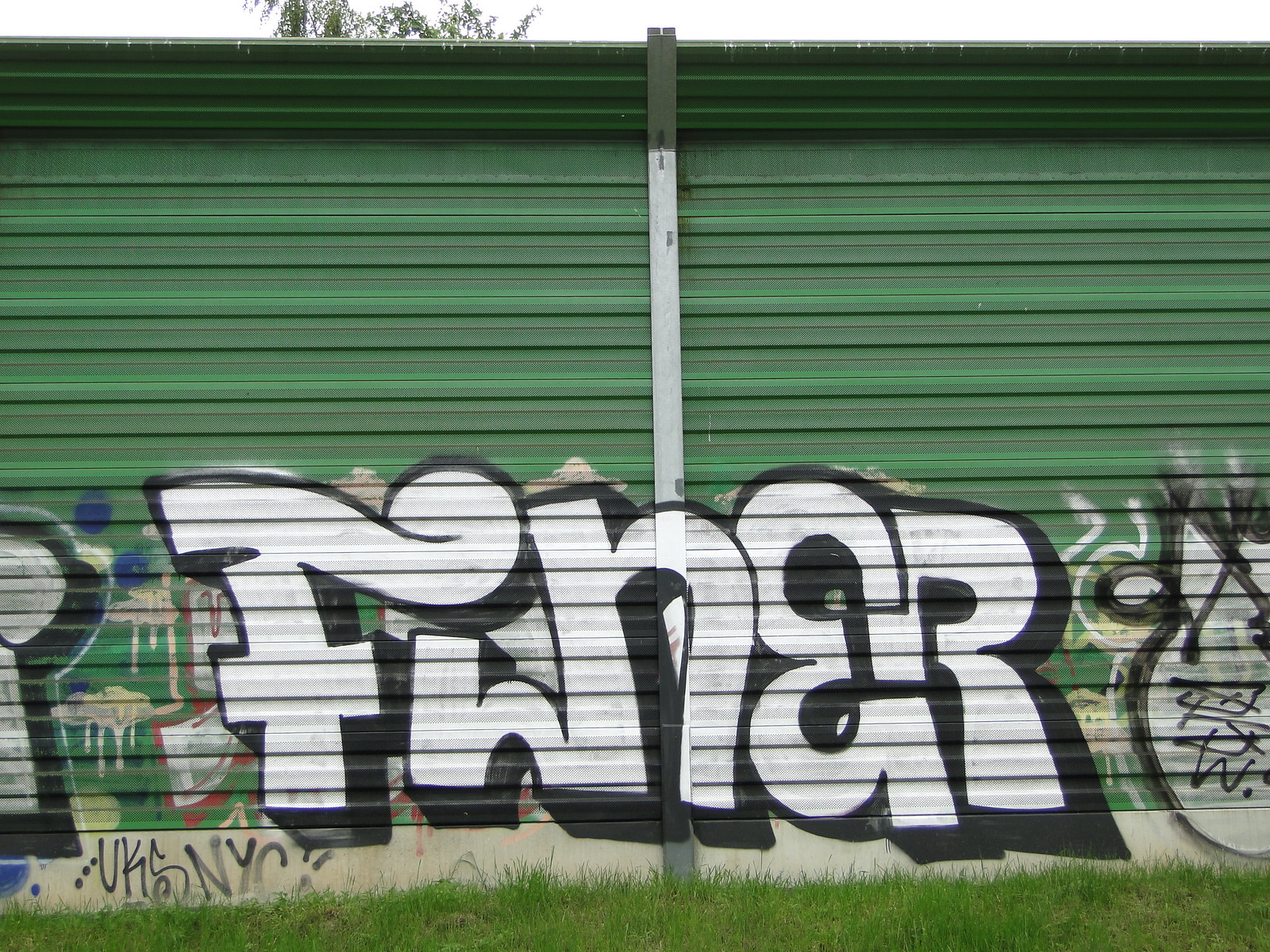In this daytime photograph, we see a green metal privacy wall adorned with graffiti, standing in an outdoor setting against a backdrop of a light gray sky. The wall features intricate sheet metal patterns that slightly curve at the top, held up by sturdy metal brackets. At the bottom half of the wall, vibrant, recently painted graffiti captures attention with prominent large, curvy white bubble letters outlined in black, likely spelling "FHNER." This fresh graffiti stands out amidst older, more worn-out tags in multiple colors such as yellow, blue, black, and additional shades of green. In the very foreground, a flat grassy area leads up to the base of the wall, while above, the top of a tree with lush green leaves peeks over, adding a touch of natural beauty to the urban scene.